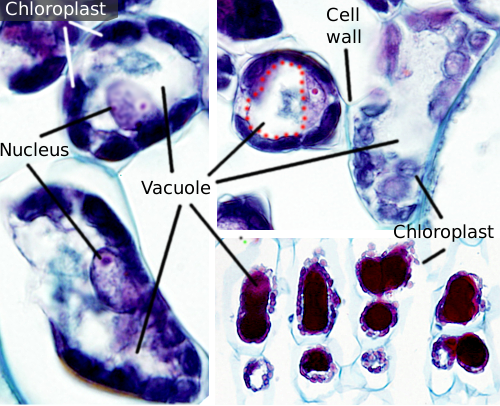The image is a detailed composite of three side-by-side microscope slides, presented in a single, vertically long, three-part photograph with a distinct white border separating each slide. Each section magnifies cells with a transparent, inky look, predominantly displaying shades of blue, purple, and hints of red. The cells have been labeled meticulously with white text and pointing lines.

On the top left corner, the word "Chloroplast" appears, pointing to the bright blue chloroplasts within the cells. Below this, "Nucleus" is labeled with lines indicating the round, purple-tinged structures. "Vacuole" is marked in the middle section with multiple lines indicating several vacuoles spread across the images, showcasing their transparent nature. The top right part of the image has a label for "Cell Wall," pointing to the cell's structural boundary, distinctly presented in blue hues. Finally, at the bottom right, "Chloroplast" appears again, this time with two lines highlighting the specific chloroplasts within the cells.

Overall, this image is a scientifically detailed illustration, likely from a laboratory setting, depicting various cell structures often seen in medical or biology textbooks, showcasing their intricate, see-through appearances magnified under a microscope.